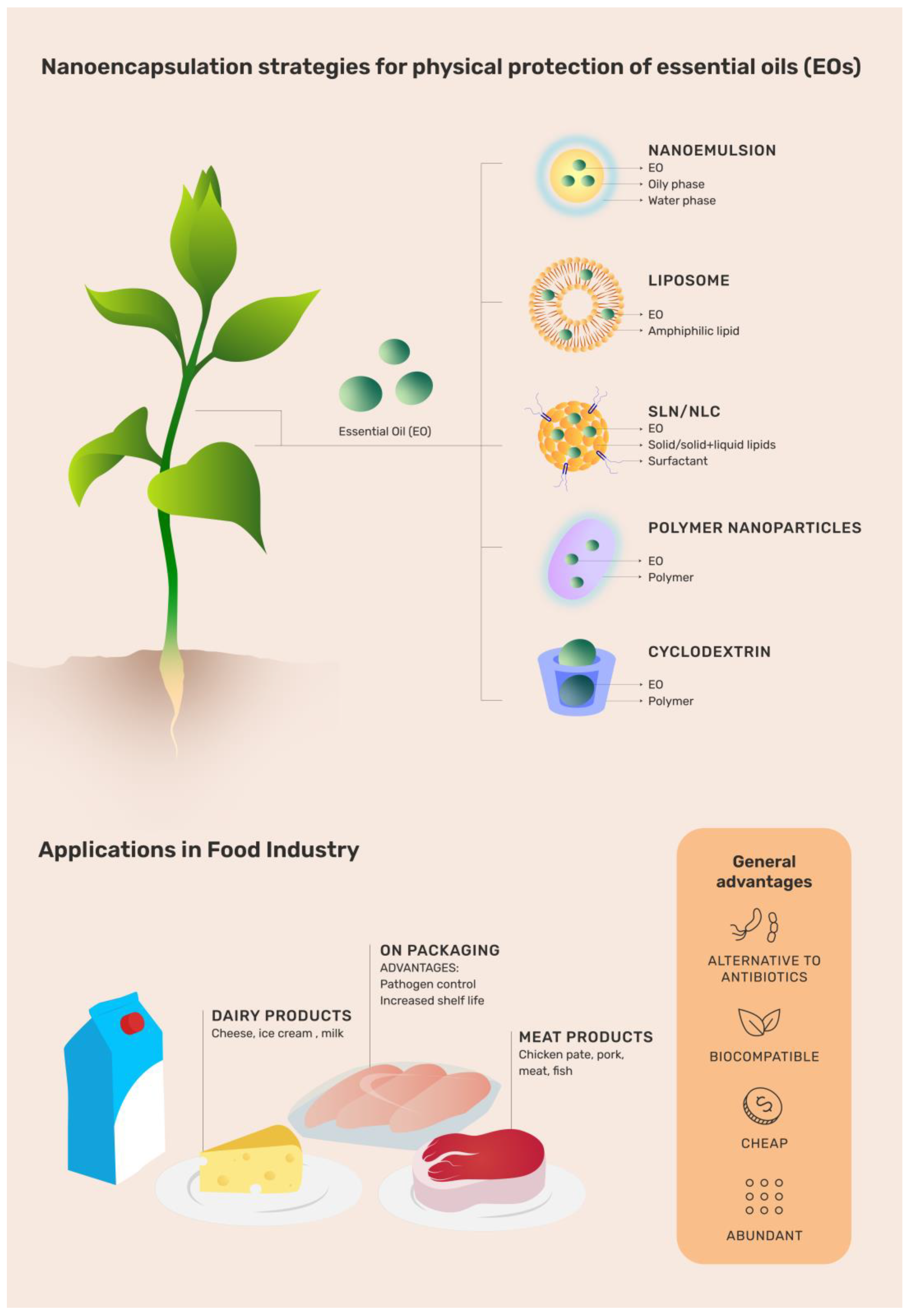The infographic depicts detailed nano-encapsulation strategies for the physical protection of essential oils, specifically tailored for the food industry. The vertical, educational-style graphic features a light brown background and is divided into two sections. The top half showcases a green, leafy plant symbolizing the source of essential oils, titled “Nano-encapsulation strategies for physical protection of essential oils.” Adjacent to it, a bracket details various encapsulation methods including Nano-emulsion, Liposome, SLN/NLC, Polymer Nanoparticles, and Cyclodextrin, each accompanied by corresponding icons.

The bottom half of the graphic is dedicated to the practical applications of these encapsulation strategies within the food industry. Illustrated items such as a milk container, cheese plate, and steak plate denote the usage of essential oils in dairy products (milk, cheese, ice cream), meat products, and food packaging. Highlighted benefits of these applications include pathogen control, increased shelf life, and alternatives to traditional preservatives. A distinctive orange text box on the bottom right outlines the general advantages of using nano-encapsulated essential oils: they serve as alternatives to antibiotics, are biocompatible, cost-effective, and abundantly available.